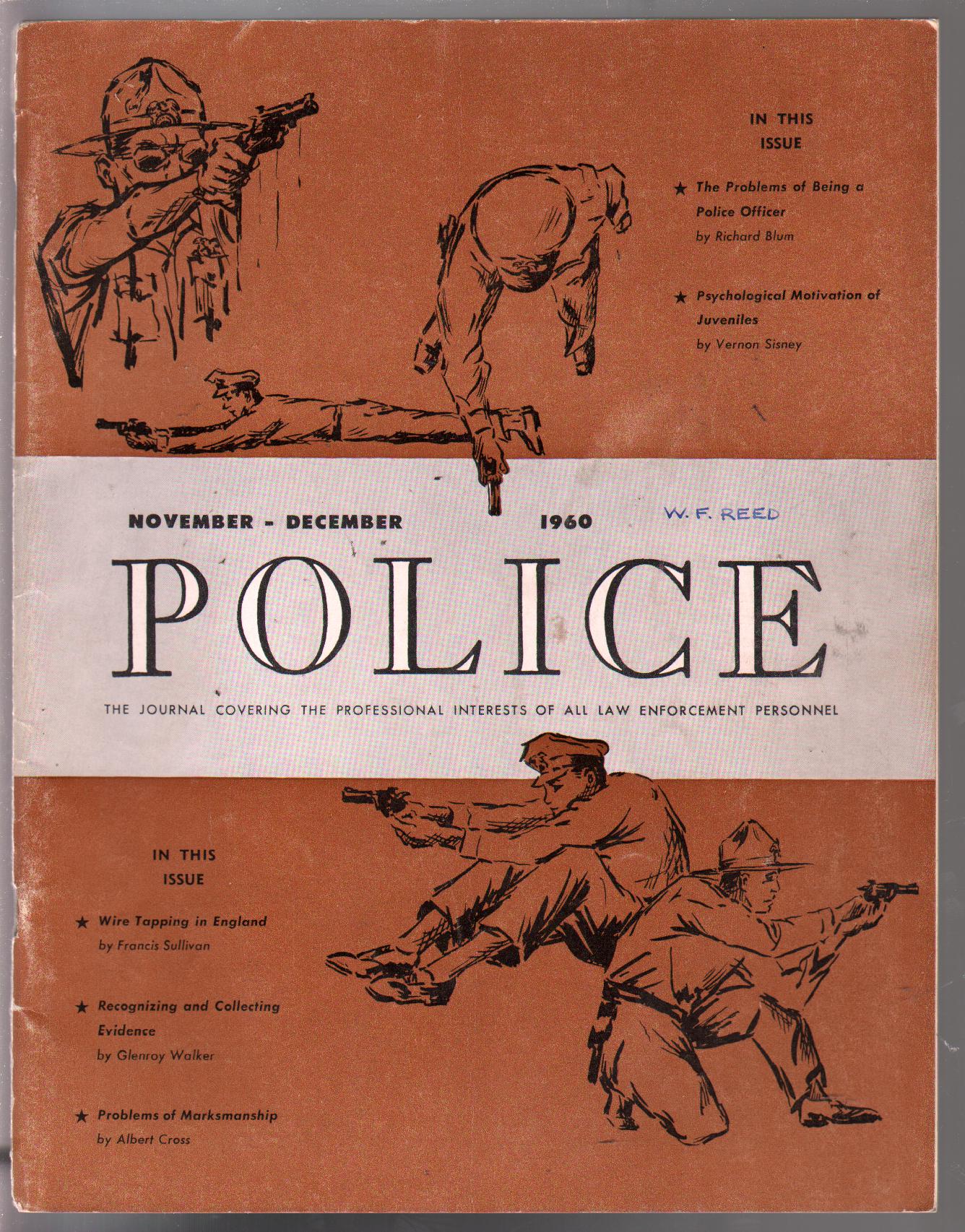The image is a full-color photograph of the cover of a vintage magazine from November and December 1960. The magazine is titled "Police: The Journal Covering the Professional Interests of All Law Enforcement Personnel." The cover is predominantly an orangish color with a coral-colored bar running through the center where the name W.F. Reed is written. The layouts feature several black illustrations of policemen in various stances, each pointing their guns. From the top left, one policeman is seen holding and pointing a gun directly at the viewer, followed by another officer laying down and aiming his weapon. An overhead shot depicts a policeman pointing his gun, and at the bottom, there are two more officers, one sitting and the other kneeling and crouching with their pistols aimed. The magazine teases articles titled "The Problems of Being a Police Officer" by Richard Blum, "Psychological Motivation of Juveniles" by Vern Sinway, and covers topics such as wiretapping in England, recognizing and collecting evidence, and the problems of marksmanship. The cover is set against a brown background.